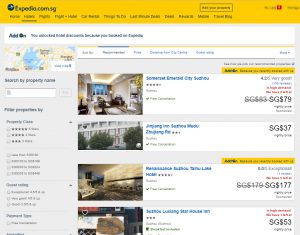The image displays a blurry webpage from Annexpedia.com. The top section features the iconic Expedia logo against a yellow bar, accompanied by the text "SG." Directly beneath the logo, there's a navigation bar, which seems to include an option labeled "add-on." Within the page, several informational sections and clickable options are visible. On the left side, there's a filter section, albeit currently empty. The main content area presents three options, each represented by an image. The first image appears to showcase a room interior, the second an exterior shot of a building, and the third likely another interior scene. Some parts of the page, specifically around the prices, are highlighted in red, while the names of the listings are prominently displayed in blue. Despite the blurriness, these elements indicate a detailed listing and filtering interface typical of travel booking sites like Expedia.